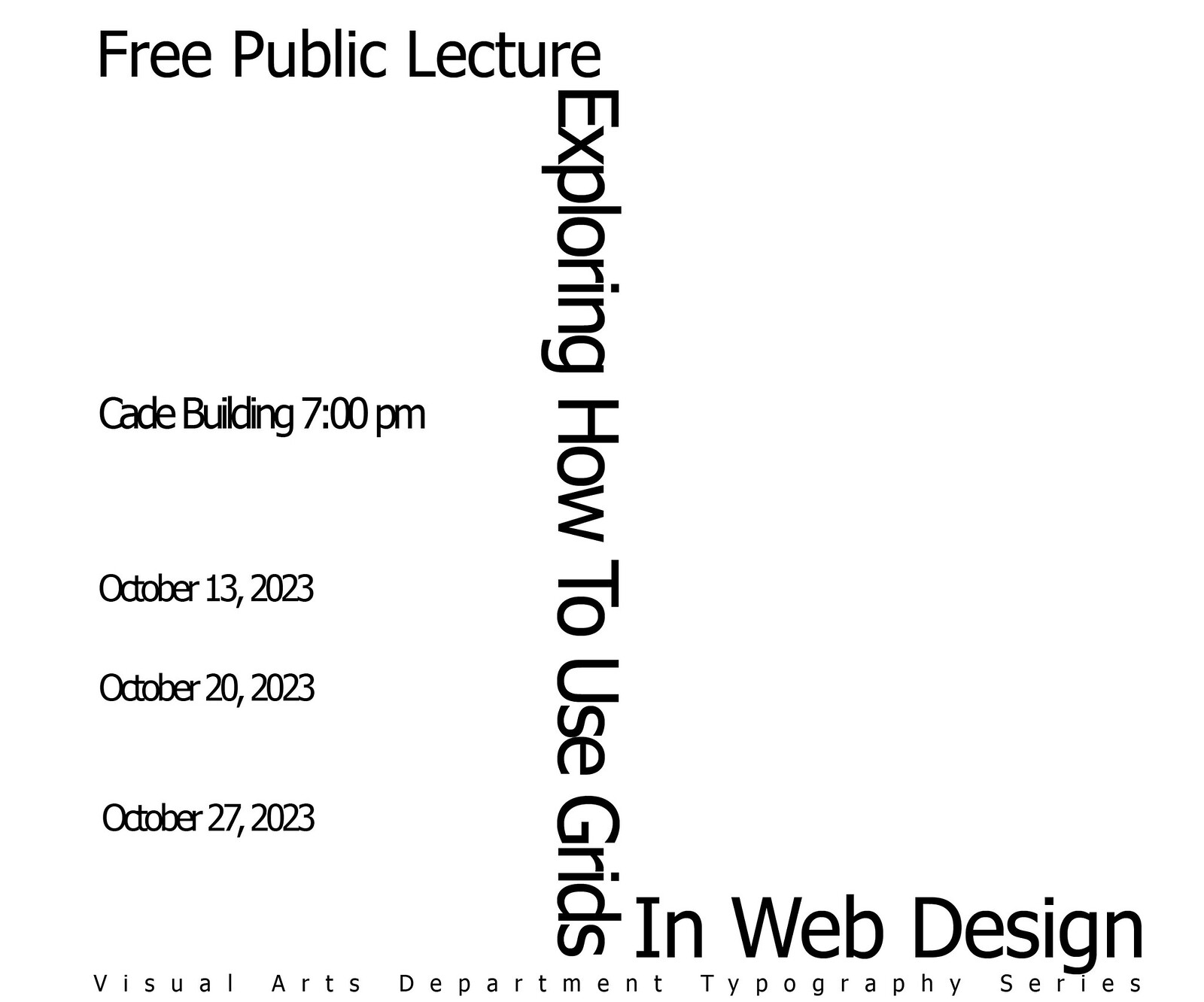This poster, rendered in a stark black and white design, advertises a free public lecture series titled "Exploring How to Use Grids in Web Design". The top left of the poster prominently features the announcement "Free Public Lecture" in bold black text. Vertically aligned in dark black lettering along the left edge, the text reads "Exploring How to Use Grids," while horizontally positioned at the bottom in the same bold style, it concludes with "in Web Design". 

On the left half of the flyer, the location "Cade Building" is noted, with the time "7 p.m." positioned below it. The dates for the lectures are listed with generous spacing as follows: October 13th, 2023, October 20th, 2023, and October 27th, 2023. Below these details and in smaller text, the statement "Visual Arts Department Typography Series" is included, indicating the organizing body of the event.